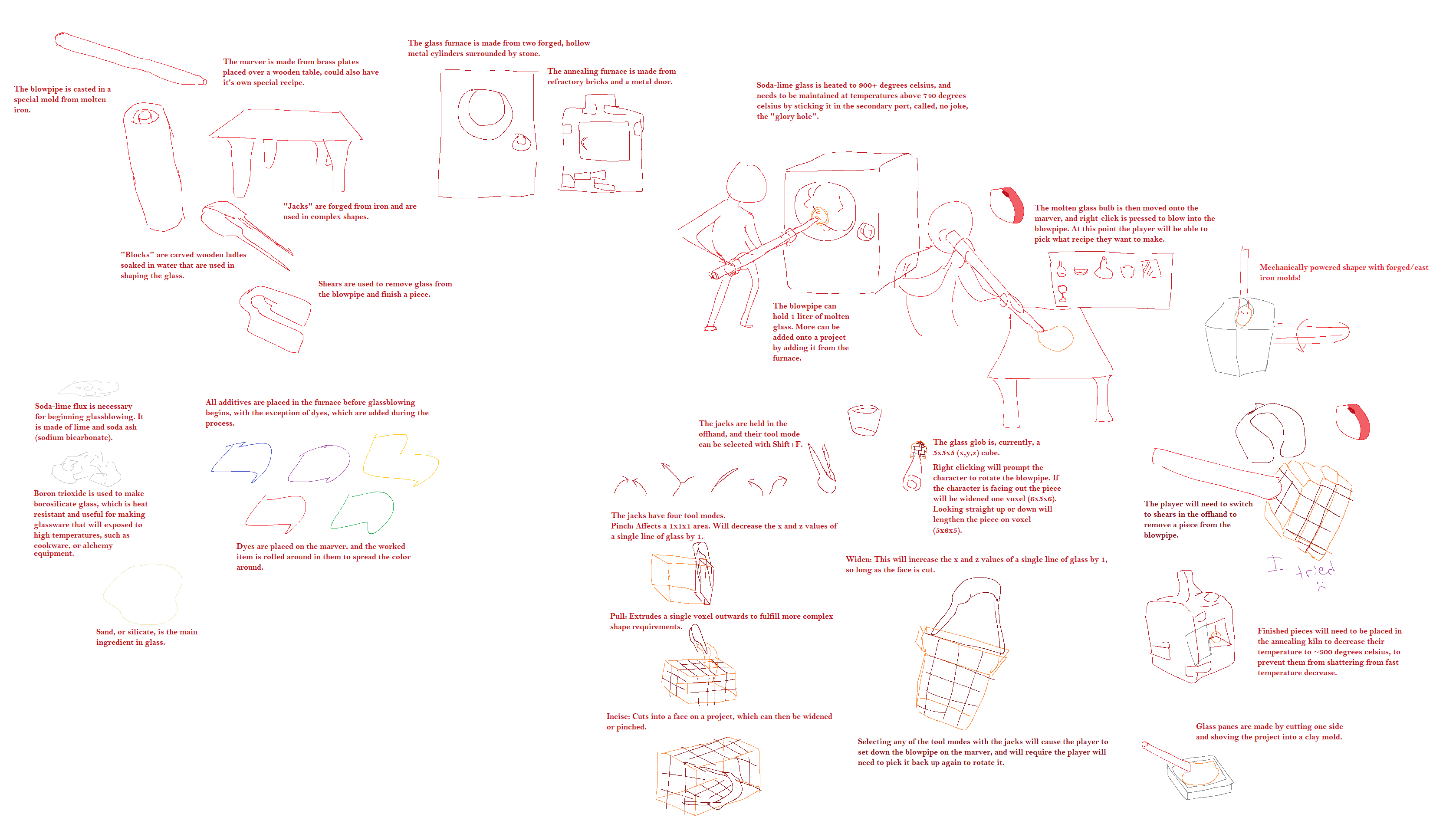This detailed caption encapsulates information from all three sources:

This image is a large rectangular informational graphic set against a white background. It features numerous amateurish, red-colored diagrams and text. The prominent elements include diagrams of a table with uneven lines, a washing machine, a television, assorted cooking utensils, an ice cream cone, boxes (some appearing three-dimensional like cubes), a metal door, and a basket with lines through it. There are also figures depicted as thick stick figures—one standing next to a clothes dryer and another seated at a table. Despite containing various explanatory images and tiny text, the purpose of the diagram remains unclear due to the illegibility and child-like quality of the drawings.